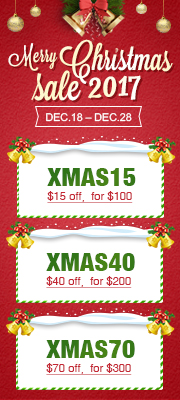The image is a vertical display ad designed for a website, celebrating Christmas with a festive theme. With dimensions about two and a half times taller than it is wide, the ad features a vibrant red background. At the top corners, left and right, there are exquisite gold Christmas tree ornaments that resemble either high-quality photos or very detailed drawings. Centered at the top is a pair of gold Christmas bells adorned with a striking red bow.

Below the bells, in elegant white calligraphy, the message "Merry Christmas" stands out, followed by "Sale 2017" in the same decorative script. Underneath, in all capital letters, the ad announces the promotional dates: "December 18th through December 28th."

Further down, the ad features three rectangular sections that resemble coupons, each highlighted with a narrow, green-and-white striped border. Each coupon shares the same visual design, featuring the gold Christmas bells with the red bow at the upper left and right corners.

- The first coupon at the top reads "XMAS15" in large green capital letters, offering "$15 off for $100" marked in red beneath it.
- The middle coupon follows suit with "XMAS40," offering "$40 off for $200."
- The bottom coupon states "XMAS70," providing "$70 off for $300."

Overall, the ad combines festive holiday elements with clear promotional offers, effectively capturing the spirit of Christmas.